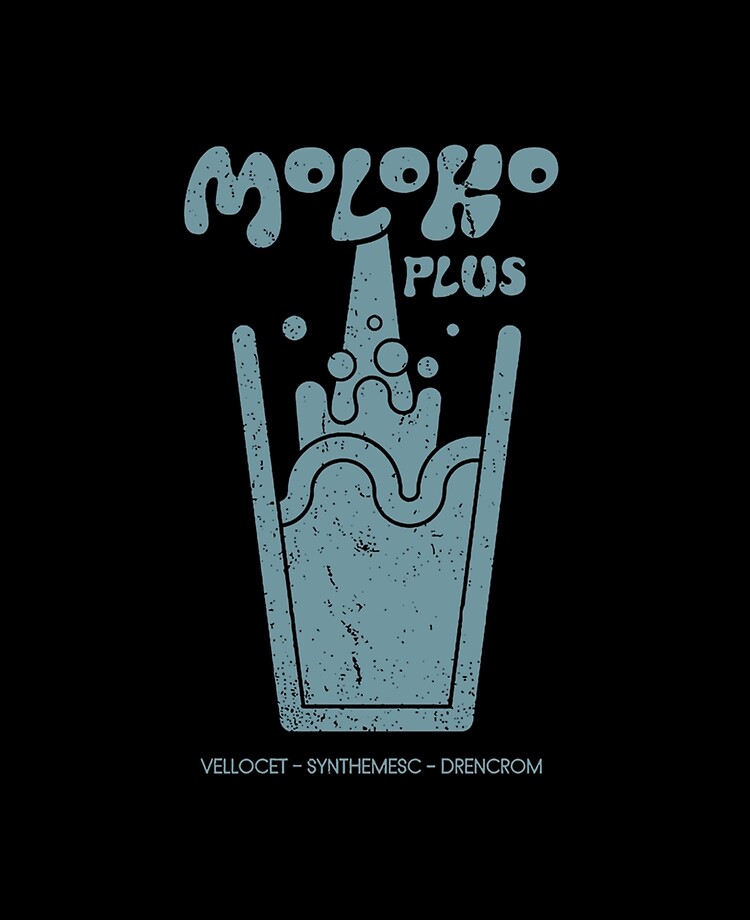The image is a distinct graphic set against a black background, reminiscent of artwork for a t-shirt or poster. At the top, the text "Moloko Plus" is displayed in playful, circular, bubble-like letters with a bluish-grey hue. The letters 'M,' 'L,' and 'K' are larger, while the 'O's are smaller and appear as superscripts, forming a visual that resembles eyes and a nose, with the 'L' taking on the shape of a nose.

Beneath this text, a light blue liquid seems to pour from the bottom of the 'L' into a stylized glass that expands as it ascends, with waves and bubbles within to indicate the presence of the liquid. This creates a splash effect dramatically reaching up to the initial 'L' in "Moloko." Below the glass, in small, similar bluish-grey text, are the foreign words: "Velocet," "Synthemesc," and "Drencrom," each separated by hyphens. This amalgamation of artistic details creates an intriguing and visually stimulating image.